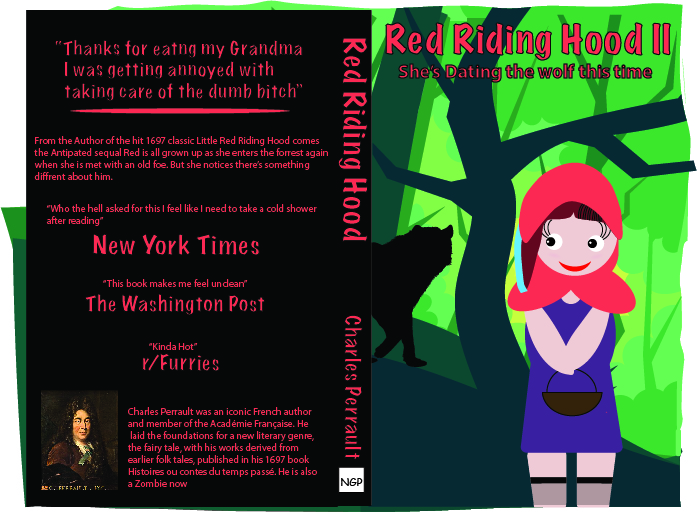The image depicts a parody e-book cover titled "Red Riding Hood 2: She's Dating the Wolf This Time." On the right-hand side, there's an illustrated front cover featuring Red Riding Hood—a girl with dark red hair, a red hat tied in a bow under her chin, gray and green socks, and carrying a black bucket—standing in a green forest with a looming tree. A shadowy figure of a wolf approaches from the left. The title "Red Riding Hood 2" is emblazoned at the top in red font, with the subtitle "She's Dating the Wolf This Time" just below.

The center seam of the image reveals the book's spine, which also reads "Red Riding Hood by Charles Perrault." Moving to the left-hand side, the back cover is set against a black background and contains a series of satirical quotes in red text. At the top, a quote says, "Thanks for eating my grandma. I was getting annoyed with taking care of the dumb bitch." Below that, promotional text reads, "From the author of the hit 1697 classic Little Red Riding Hood comes the anticipated sequel. Red is all grown up as she enters the forest again where she is to meet with an old foe. But she notices there's something different about him." 

Critiques follow, with exaggerated reviews like, "Who the hell asked for this? I feel like I need to take a cold shower after reading," attributed to the New York Times, and "This book makes me feel unclean," from the Washington Post. Another humorous review from "R/ Furries" says, "It's kinda hot." At the bottom left corner of the back cover, there is a painting of the author, accompanied by his quirky biography: "Charles Perrault was an iconic French author and member of the Académie Française. He laid the foundation for a new literary genre, the fairy tale, which is derived from earlier folktales published in his 1697 book Histoires ou Contes du Temps Passé. He’s also a zombie now." This satirical e-book cover merges classical references with modern, dark humor.